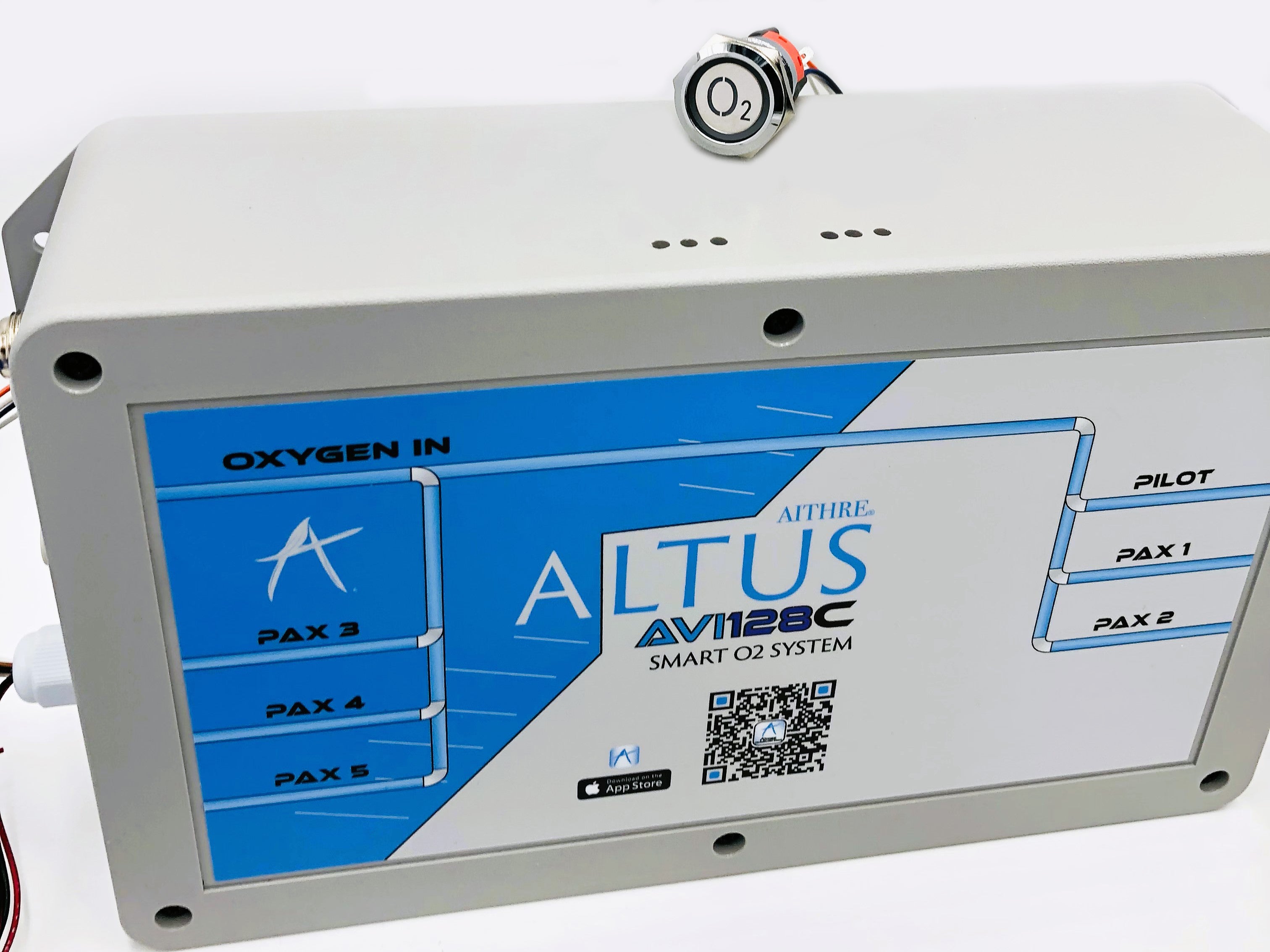The image depicts the Altus AVI28C Smart O2 System, a grayish or white aluminum box equipped with various features indicating its function as an oxygen management unit. The box has a blue and white label on the front and includes a handwritten logo with the Altus branding. There are multiple indicator lights and labels such as "Oxygen In," "Pax 3," "Pax 4," "Pax 5," and "Pilot" with "Pax 1" and "Pax 2," suggesting different segments or packs associated with the unit. Right side indicators and ports imply connectivity options with external devices or systems, and numerous wires can be seen plugged into the unit. On top of the box, there's a button labeled "O2" and what appears to be an oxygen measuring watch resting on it. Additionally, there is a QR code printed on the unit, likely for quick information access. The precise purpose of the device is ambiguous, but details suggest it's used for controlling or measuring oxygen, potentially in a sophisticated filtration or air management context.